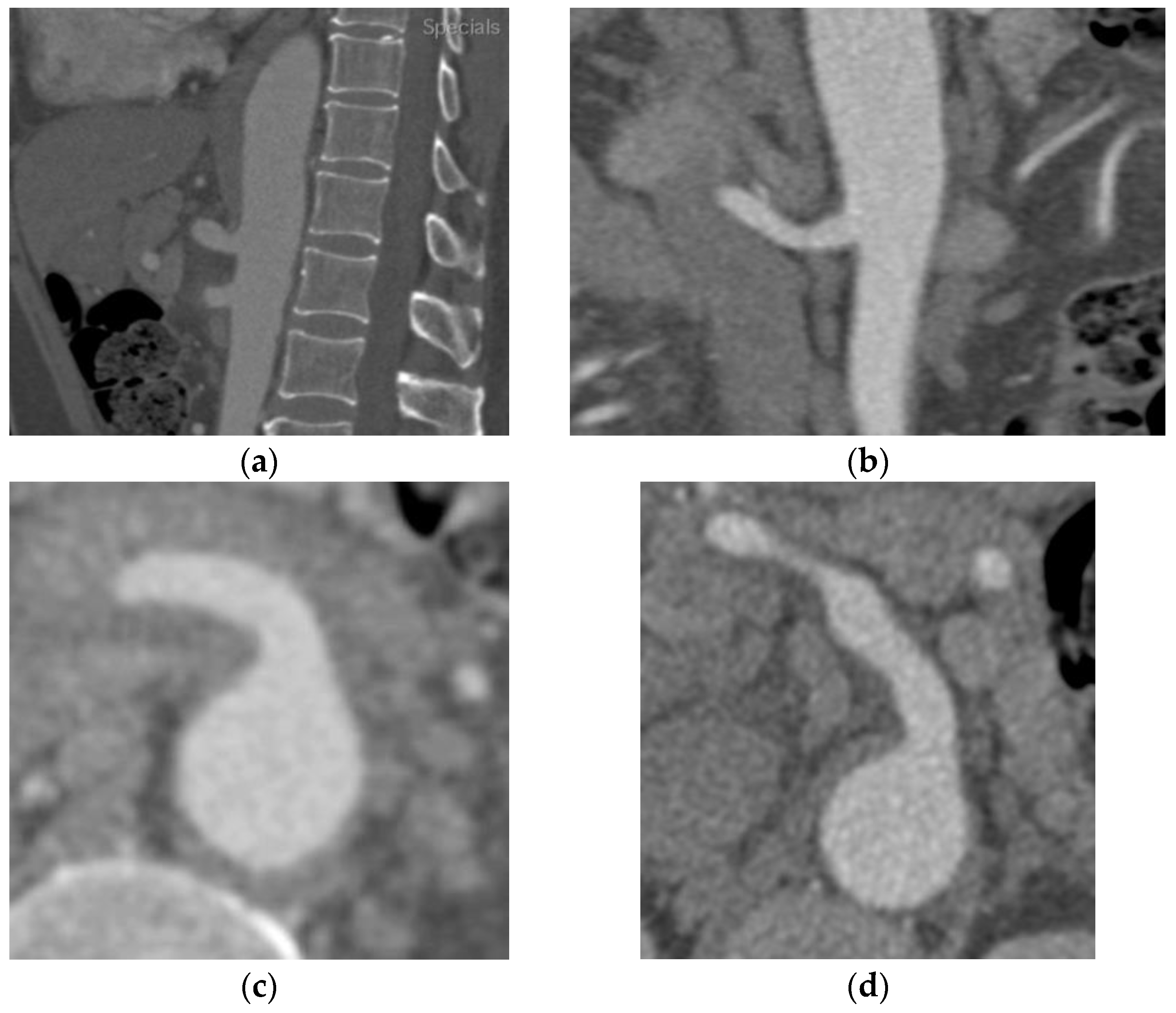The image is divided into four sections labeled A, B, C, and D. Each section contains a black and white, possibly x-ray photograph, with images in shades of grey. The top left image, A, appears to be an x-ray of a segment of the spine, clearly showing individual vertebrae. To the left of the spine in A, there is a white, oval-like shape with two smaller protrusions, resembling feet. The top right image, B, seems to be a zoomed-in x-ray focusing on internal organs, with a blob-like structure that may include a hand and an appendage or thumb. The bottom left image, C, further zooms into a rounded, comma-shaped object, resembling a vertically reversed number 6. Finally, the bottom right image, D, shows the most zoomed-in view of what appears to be an elongated comma shape, continuing the pattern of internal structure exploration. All the images share a slightly blurry quality, potentially indicating a microscopic or radiographic technique.